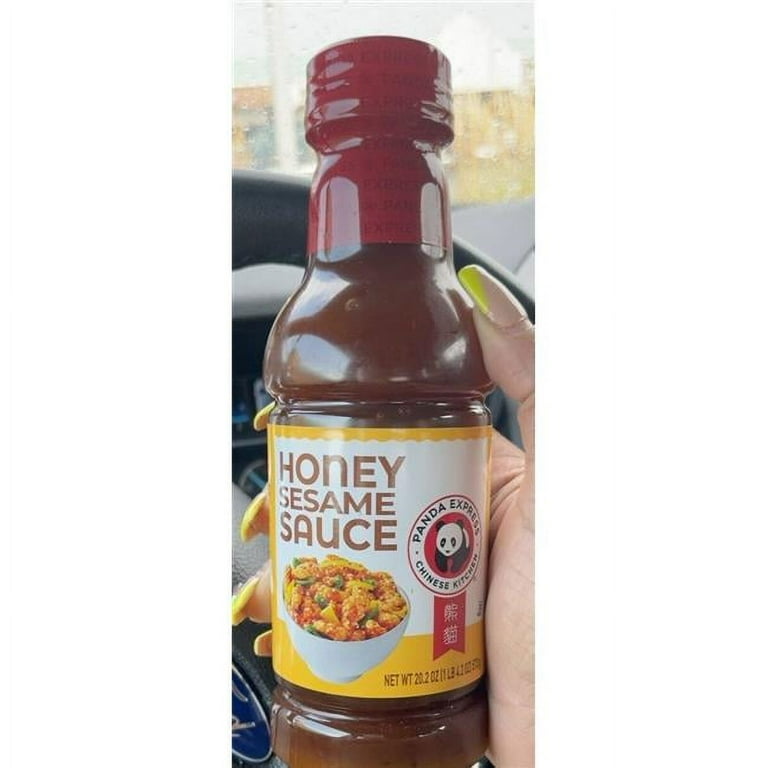This detailed photograph captures a Caucasian hand adorned with long, acrylic nails that have bright neon yellow and neutral nude tips, holding a plastic bottle of Panda Express Honey Sesame Sauce. The sealed bottle, featuring a red shrink-wrapped cap, contains a dark brown sauce. The bottle’s label is distinctly designed with a gold outline and brown text on a white background, prominently reading "Honey Sesame Sauce." A depiction of a white bowl filled with fried rice and vegetables, paired with the recognizable Panda Express logo featuring a panda, completes the bottle’s presentation. The scene is set inside a Ford vehicle, visible by the steering wheel and partial logo, with a blurred background of buildings seen through the windshield, suggesting the vehicle is parked. This meticulously staged photo emphasizes the product prominently while providing context through its setting.